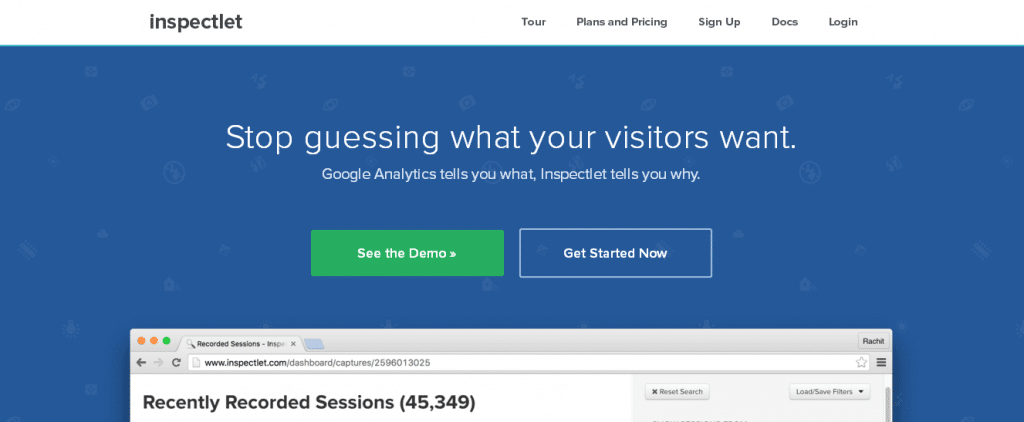The screenshot captures the top edge of a laptop screen, characterized by a wide yet narrow display. At the very top, the text reads "Inspectlet," followed by navigation options including "Tour," "Plans and Pricing," "Sign Up," "Docs," and "Login." The main background appears blue-green, featuring the text: "Stop guessing what your visitors want. Google Analytics tells you what, Inspectlet tells you why." Below this text, there are two prominent buttons: a green one labeled "See the Demo" and another to the right labeled "Get Started Now."

Additionally, a pop-up window overlays the background. This smaller window, headlined "Recently Recorded Sessions 45,349," shows a reduced version of the screen and the URL "www.inspectlet.com." The overlay screen partially obscures the blue-green main screen, presenting a detailed, layered view of the Inspectlet interface.